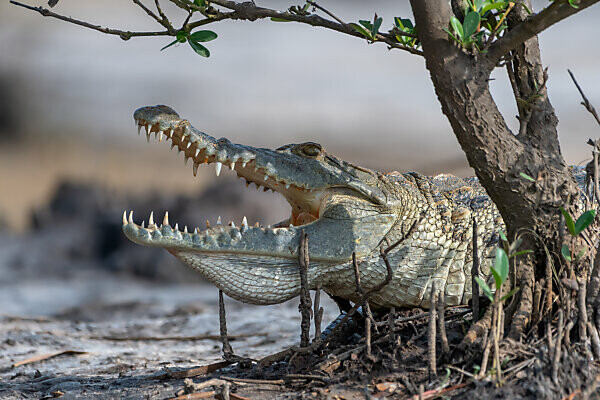This is a photograph of a menacing alligator emerging from behind a tree on the right-hand side of the image. The alligator, with its mouth wide open, showcases rows of sharp, white, conically shaped teeth. Its scaly skin exhibits a dull gray-green coloration, with hints of cream and black interspersed. One dark black eye is visible above its gaping mouth, giving it an alert and ferocious look. The gator's head and mouth are pointed towards the left side of the image. Surrounding the alligator, a few green leaves are observed on the branches of the tree. The background is a blurred mixture of light gray, beige, and orange hues, with a fuzzy appearance that emphasizes the focus on the alligator and the tree, reminiscent of a swamp or possibly a dry river basin.